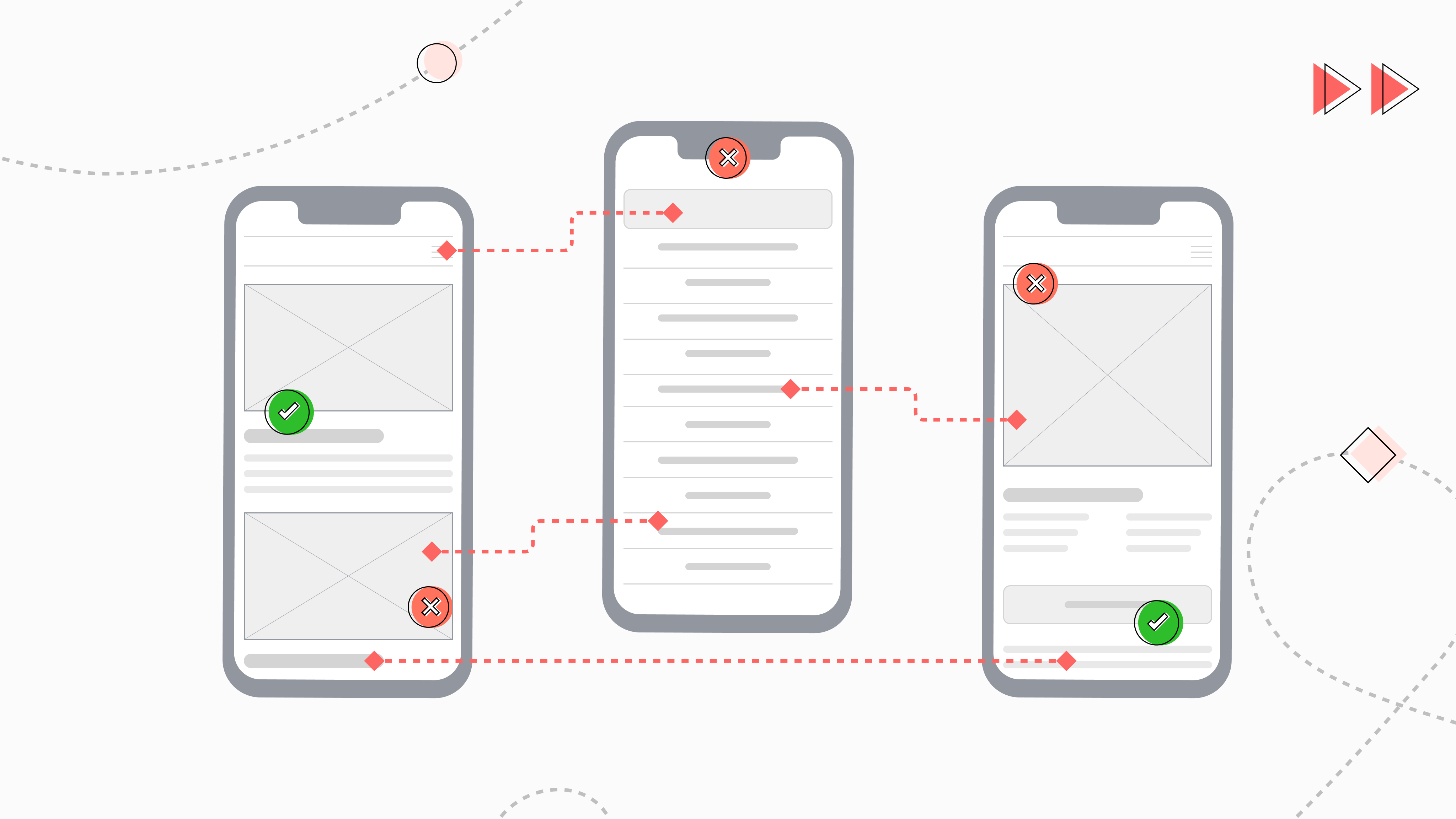The image depicts a hand-drawn, minimalistic diagram of three iPhone-like cell phones arranged in a horizontal sequence. The phones are separated equally, with the center phone positioned slightly higher than the other two. Red arrows with dots and hyphenated lines connect each of the phones, forming a flowchart-like design. On the first phone (left), there's a green check mark in a circle at the top middle, indicating the correct action, and a red X at the bottom right, signaling an incorrect action. The second phone (center) features a red X at the top, marking another incorrect action. The third phone (right) has a red X at the top and a green check mark at the bottom, suggesting the final correct action. The recurring symbols and connections imply the diagram is instructional, possibly illustrating the correct and incorrect steps for an email process or page navigation on a cell phone.